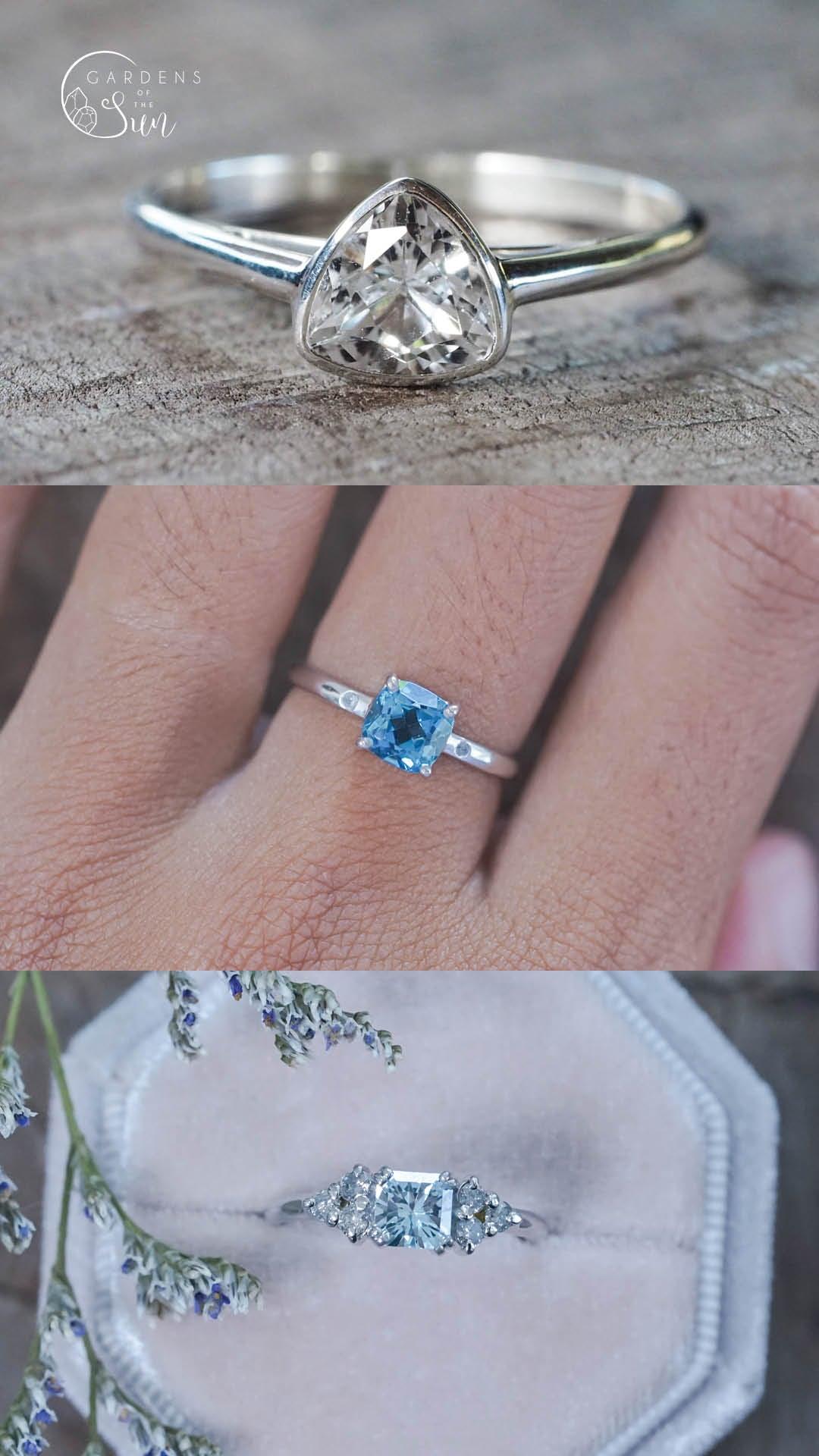This photorealistic triptych advertisement showcases three distinct engagement rings, emphasizing their unique characteristics and settings. The top panel features a heart-shaped clear diamond ring set in silver, elegantly displayed on a wooden table with the logo "Gardens of the Sun" overhead. The center image captures a gold ring with a square-cut sapphire on a woman's hand, highlighting the sapphire’s deep blue hue. The bottom panel presents a diamond ring with a subtle hint of blue, nestled in a pale blue, satin-lined jewelry box. A delicate spray of forget-me-nots decorates the scene, further accentuating the ring's elegance and the store's attention to detail. This advertisement clearly aims to invoke the beauty and craftsmanship of the jewelry offered by Gardens of the Sun.